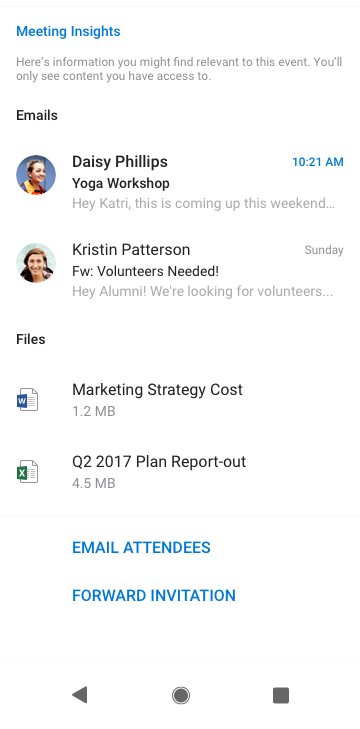A screenshot of a meetings or invitation app displays a feature called "Meeting Insights" which highlights relevant information for an upcoming event. The notification explains that users will see only the content for which they have access. 

**Emails Section:**
- **Daisy Phillips**: 
  - **Subject**: Yoga Workshop
  - **Time**: 10:21 AM
  - **Message Preview**: "Hey Katri, this is coming up this weekend."
  - **Profile Photo**: Icon of Daisy Phillips
  
- **Kristen Patterson**: 
  - **Subject**: Forward - Volunteers Needed Sunday
  - **Message Preview**: "Hey alumni, we're looking for volunteers..."
  - **Profile Photo**: Different icon than Daisy's 

**Files Section:**
- **Document 1**:
  - **Type**: Word Document, identifiable by the "W" icon on the left
  - **Title**: Marketing Strategy Cost
  - **Size**: 1.2 MB
  
- **Document 2**:
  - **Type**: Excel Document, indicated by the "X" icon
  - **Title**: Q2 2017 Plan Report/Out
  - **Size**: 4.5 MB

**Actions at the Bottom:**
- **Email Attendees** button in blue or green text
- **Forward Invitation** option
- Standard gray navigation buttons at the bottom (triangle, circle, square)

The app provides a summary of emails, linked documents, and options to interact with event attendees, suggesting an environment for organizing or attending meetings. The view shown in the screenshot appears to be scrolled down, implying there is more information available.